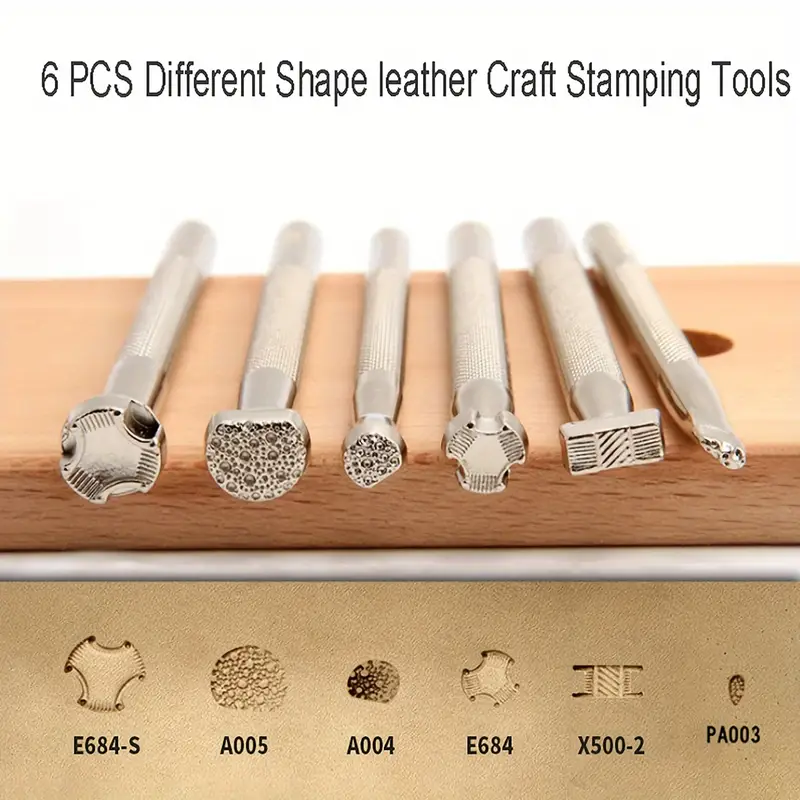This is an image showcasing a set of six silver leather craft stamping tools, each with ridged, narrow handles and distinctively shaped heads. These tools are neatly organized in custom-carved divots in a light brown wooden block, which rests atop a combination of metal surfaces. The upper section features a silver metal plate, while beneath it lies a brass-colored rectangular plate. Each tool is labeled with unique alphanumeric codes such as E684 and X502. Above these labels, the corresponding stamp patterns are displayed, illustrating the impressions these tools make on leather. For example, the round tool produces a circular imprint, another makes a pattern resembling a tiny raindrop, and others create unique shapes like diagonal-lined rectangles and variably sized geometric designs. The tools are collectively described as a "6 PCS, 6 pieces, different shaped leather craft stamping tools" in the text across the top of the image.